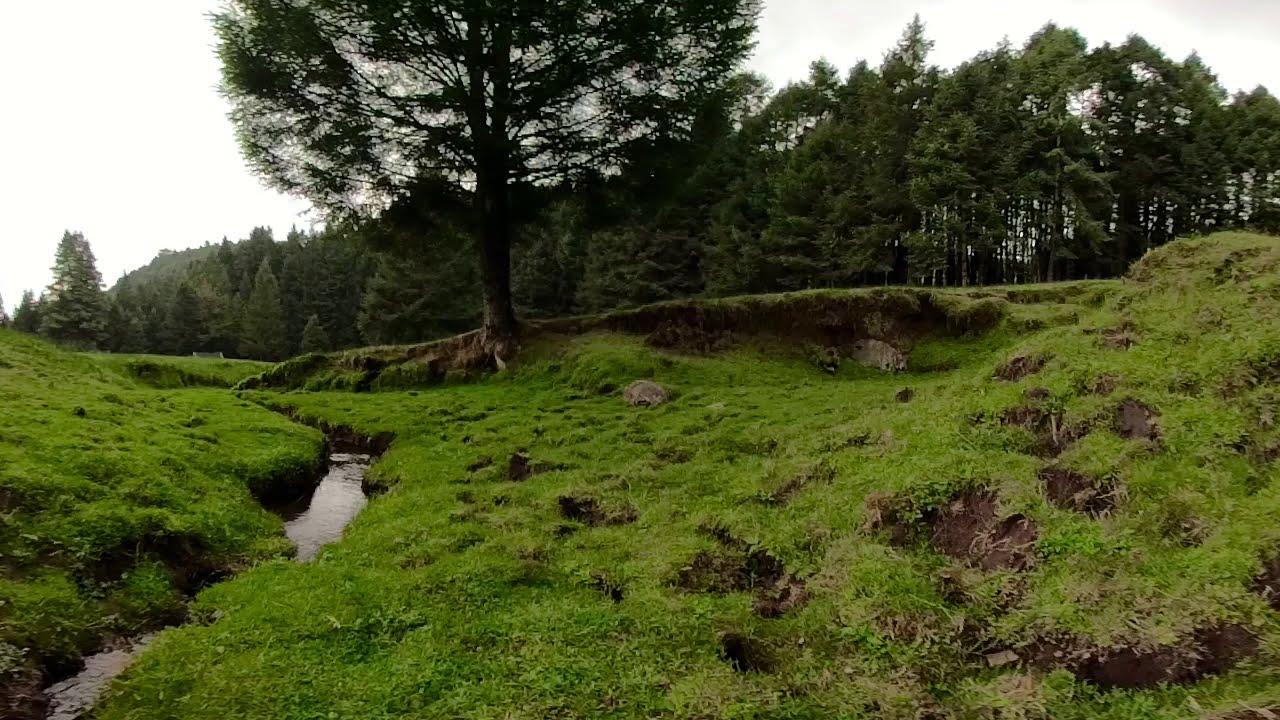The image depicts a serene countryside landscape centered around a small, meandering stream that begins in the bottom left-hand corner and curves gracefully through the scene, flanked by grassy banks. To the left of the creek, the grassy terrain gently ascends, suggesting the start of a hill. To the right of the creek, the ground is similarly grassy with scattered rocks and undulates upwards, culminating in a mixed grove of trees that extends across the upper background of the image. A prominent tree rises from a mid-ground ridge, adding a focal point. The sky is overcast, casting a diffused light across the scene, contributing to the vibrant greenery and sporadic patches of brown mud within the meadow-like foreground. Small, indistinct white objects can be seen on the far left, adding a touch of mystery to the otherwise peaceful and verdant setting.